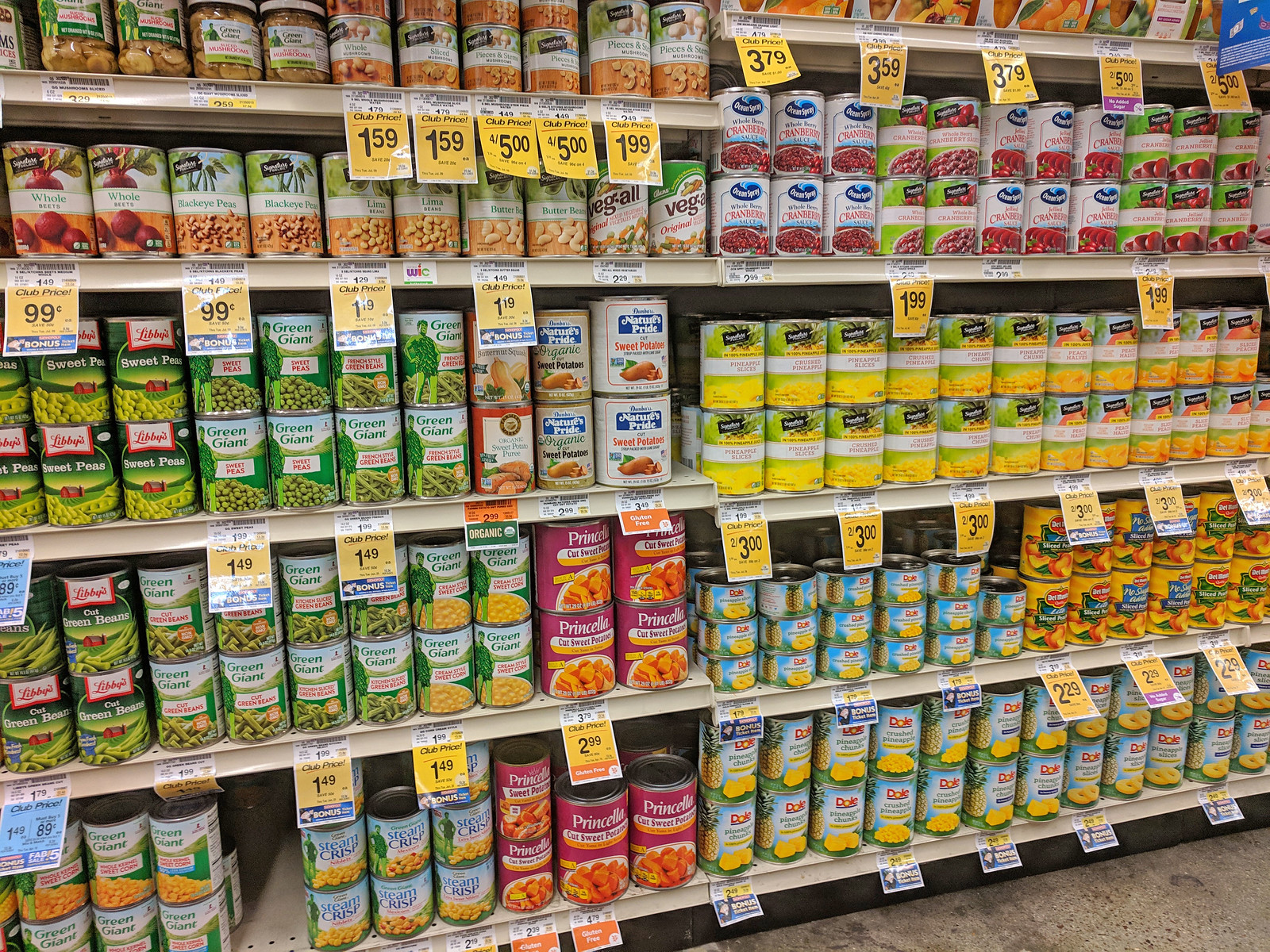The image captures a detailed view of a vegetable aisle inside a grocery store, showcasing a diverse array of products neatly displayed on four metal shelves. The shelves are stocked with a variety of vegetables, including cans of Green Giant green beans, easily recognizable by the iconic Green Giant mascot on the label. Other prominent brands include Libby's, with its distinctive red and white label, and a range of canned fruits from Del Monte and Dole. Prices are clearly marked below the items, starting at 99 cents and going up to five dollars. Despite some items being partially obstructed, the wide selection of vegetables and fruits, including cranberry sauce and pineapples, is evident, offering a comprehensive glimpse into the variety available in this grocery store aisle.